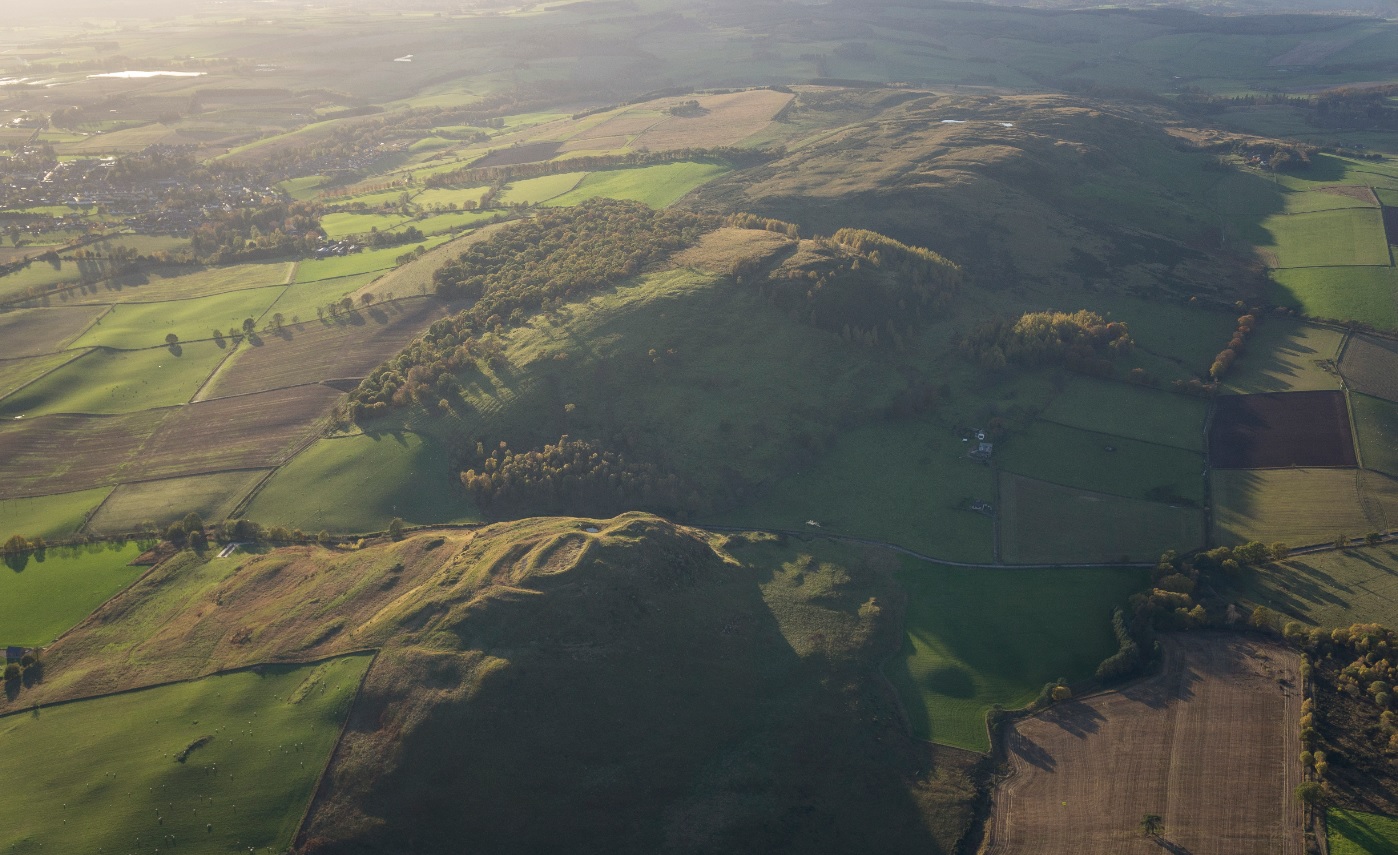This is an aerial photograph taken on a sunny, slightly hazy day, likely from a drone or an aircraft, capturing an expansive, lush landscape of rolling hills and patchwork fields in various shades of green and brown. Shadows cast from the left side suggest the sun is at an angle, elongating the shadows. The terrain features a ridge of hills running vertically through the center of the image, dotted with small trees or bushes that are not particularly tall. Scattered throughout the landscape are patches of farmland and manicured pastures, some of which appear to hold tiny white dots that might be animals, possibly cows. In the upper left corner, a denser cluster of trees and possibly some homes are noticeable, along with what looks like a body of water and a parking area. The meticulously divided plots of land give the area a quilt-like appearance, hinting at agricultural use. The overall effect is one of serene, rural beauty that might evoke thoughts of places like Ireland.